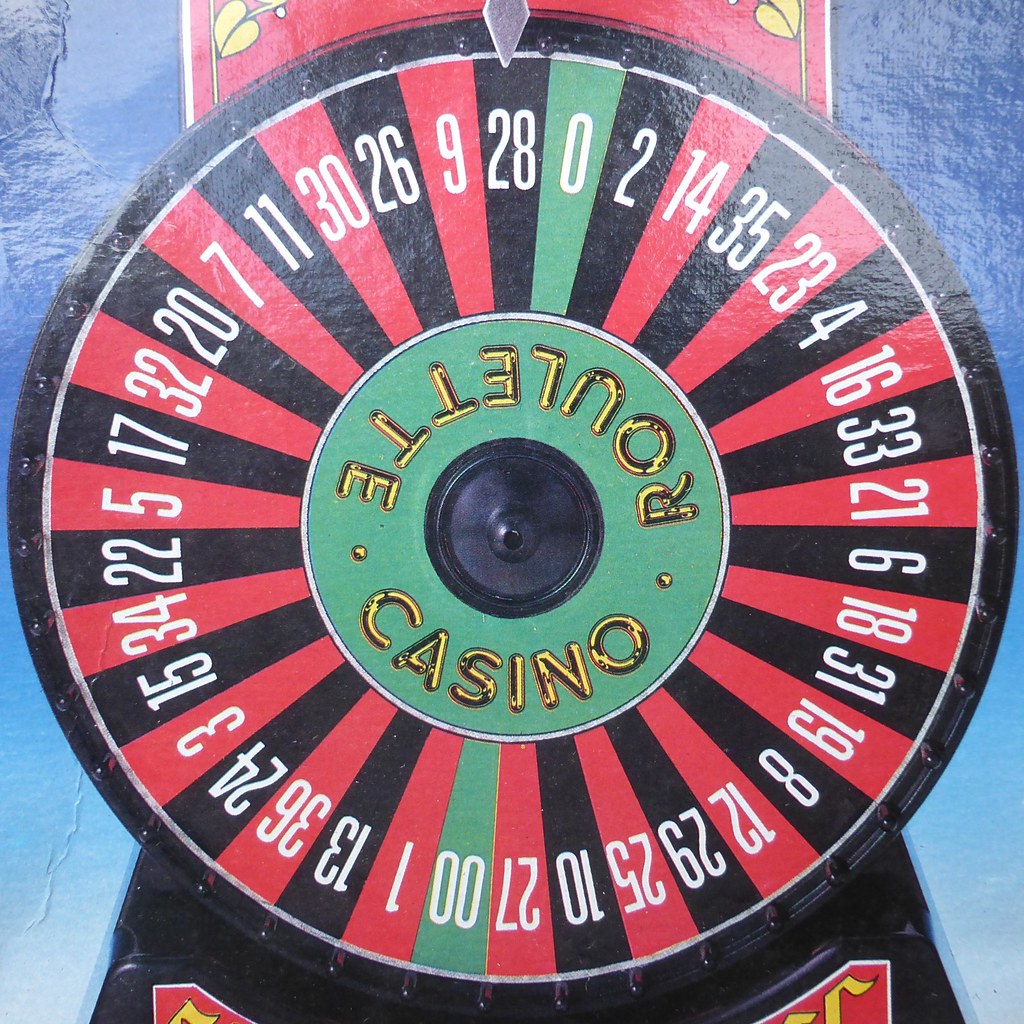The photograph showcases a central roulette wheel in a casino setting, presented against a rich blue background that transitions from dark at the top to lighter at the bottom. The wheel, which prominently features alternating red, black, and green numbered segments, stands out sharply against this backdrop. The numbers, bordered in distinct colors - red and black for the regular numbers and green for the 0 and 00 - are in white text. The wheel’s design is such that the red, black, and green colors alternate, ensuring a clear visualization for each segment. In the very center of the wheel, within a green circle, the text "Roulette Casino" is visible. Additionally, the roulette numbers are specifically laid out in a non-sequential order, with currently, the arrow pointing at the number 28 at the top of the wheel. This detailed setup epitomizes the classic allure and excitement found in a casino environment.